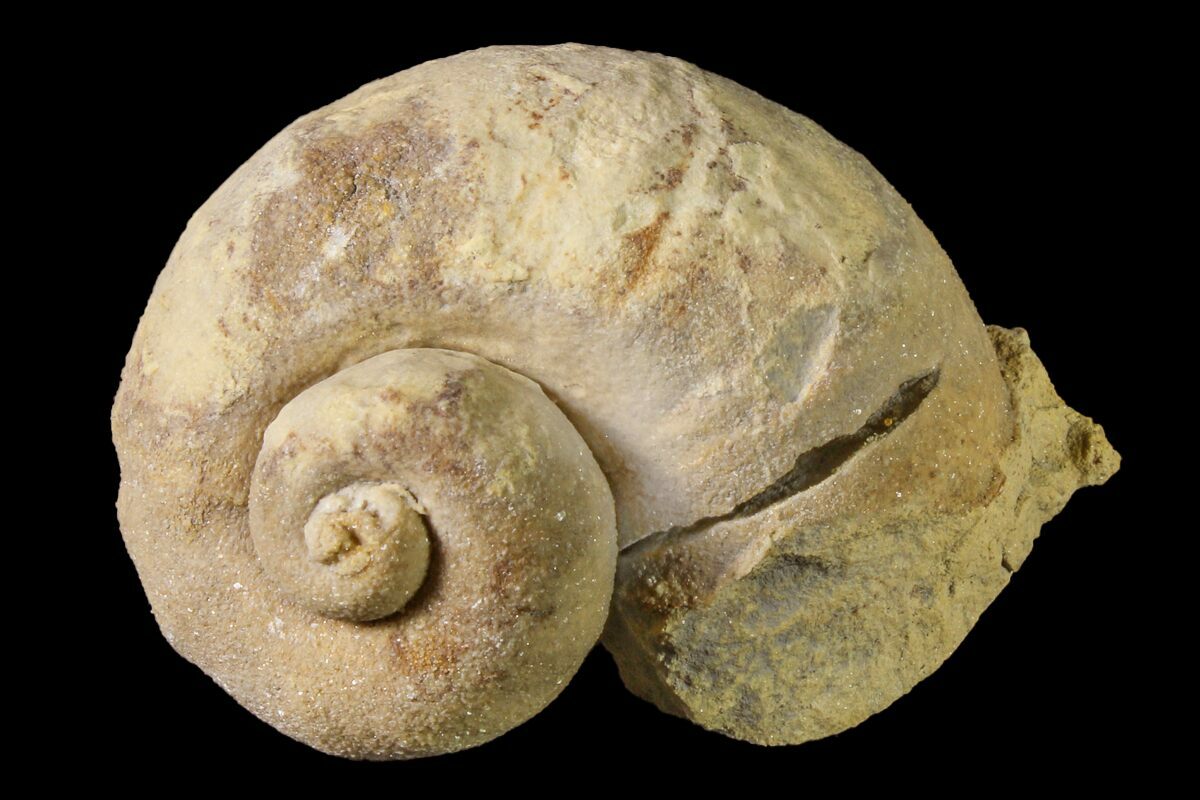The image displays an intricately detailed ancient fossil resembling a petrified snail, centered against a stark black background. This singular object, taking up most of the horizontal rectangular frame, features a spiraled shell typical of snails, with a rough and crusty texture suggestive of its age. The fossil, likely an artifact from a natural history museum exhibit, exhibits a light brown to light gray color, partially covered in earth clay material. The rounded body loops in a characteristic swirl, culminating in an open opening at the top. The upper part of the shell and some sections towards the bottom are encrusted with a lighter, crust-like material. Additionally, the structure exhibits a vaguely head-like protrusion on the right side, hinting at where a face or nose might have been, further enhancing its fossilized appearance.